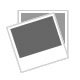The image features two clear glass jars, each with a black plastic screw-on lid. Both jars have white labels with a distinctive pink square in the middle. The jar on the left contains a metallic-looking mineral and is labeled with the periodic symbol "Sc," the atomic number "21," and the element name "Scandium." The jar on the right houses a similar type of mineral and is labeled with the periodic symbol "Y," the atomic number "39," and the element name "Yttrium." Both labels prominently display the "Nova Elements" logo in green, along with additional details about the contents. Despite slight misalignments, the label designs are consistent, with the pink squares clearly contrasting against the white background, which features black text.